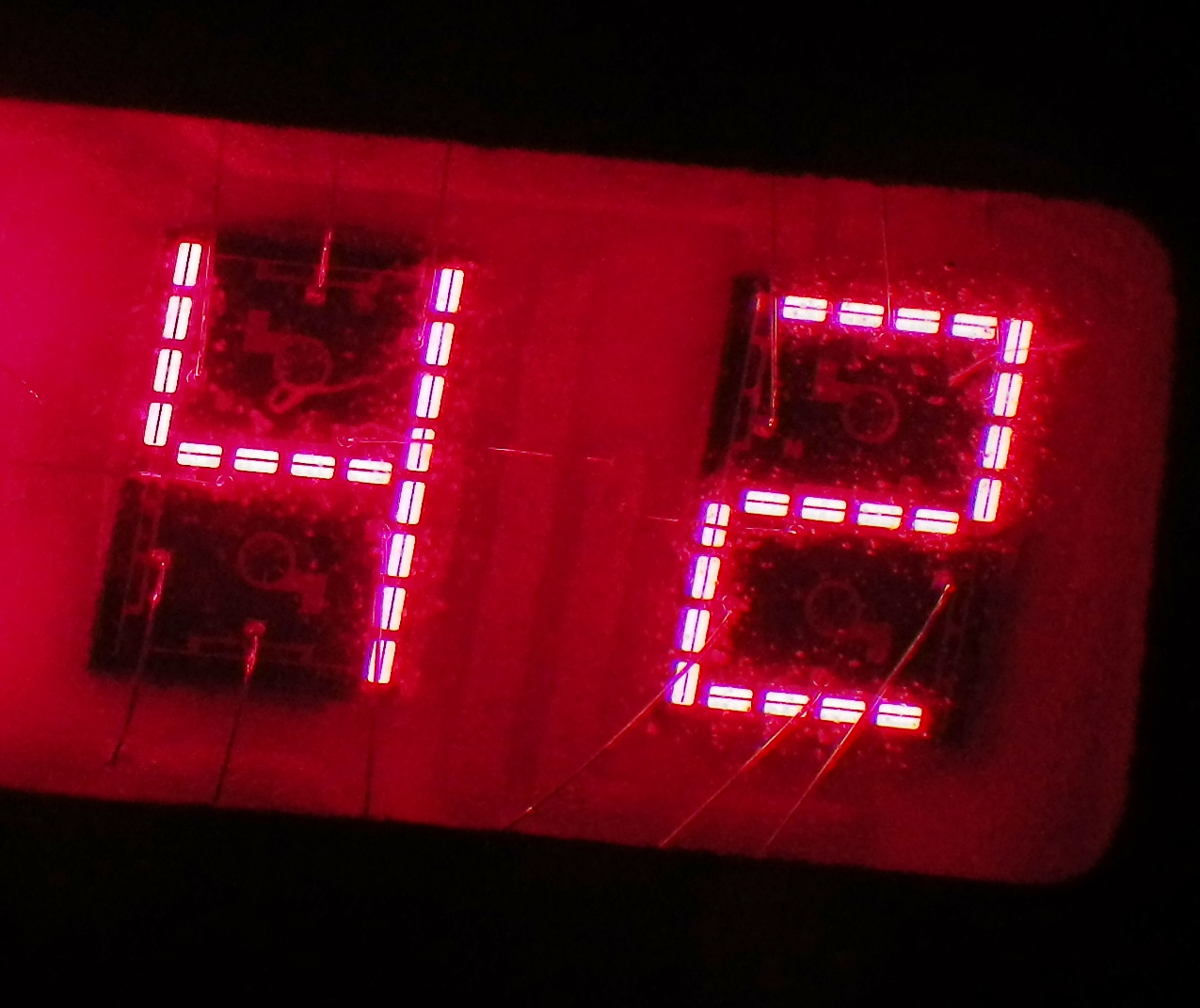In this somewhat grainy image, we observe a pitch-black background that sharply contrasts with the large red rectangular object at the center. The object appears to be a digital clock display. In crisp white digital light, the numbers "42" dominate the red face of the clock. The digits are presented in a block style, devoid of any rounded edges. Each numeral is composed of small illuminated rectangular segments that connect to form the numbers "4" and "2." Beneath and to the right of these numbers, the red face of the clock features a shaded area, adding depth to the display.